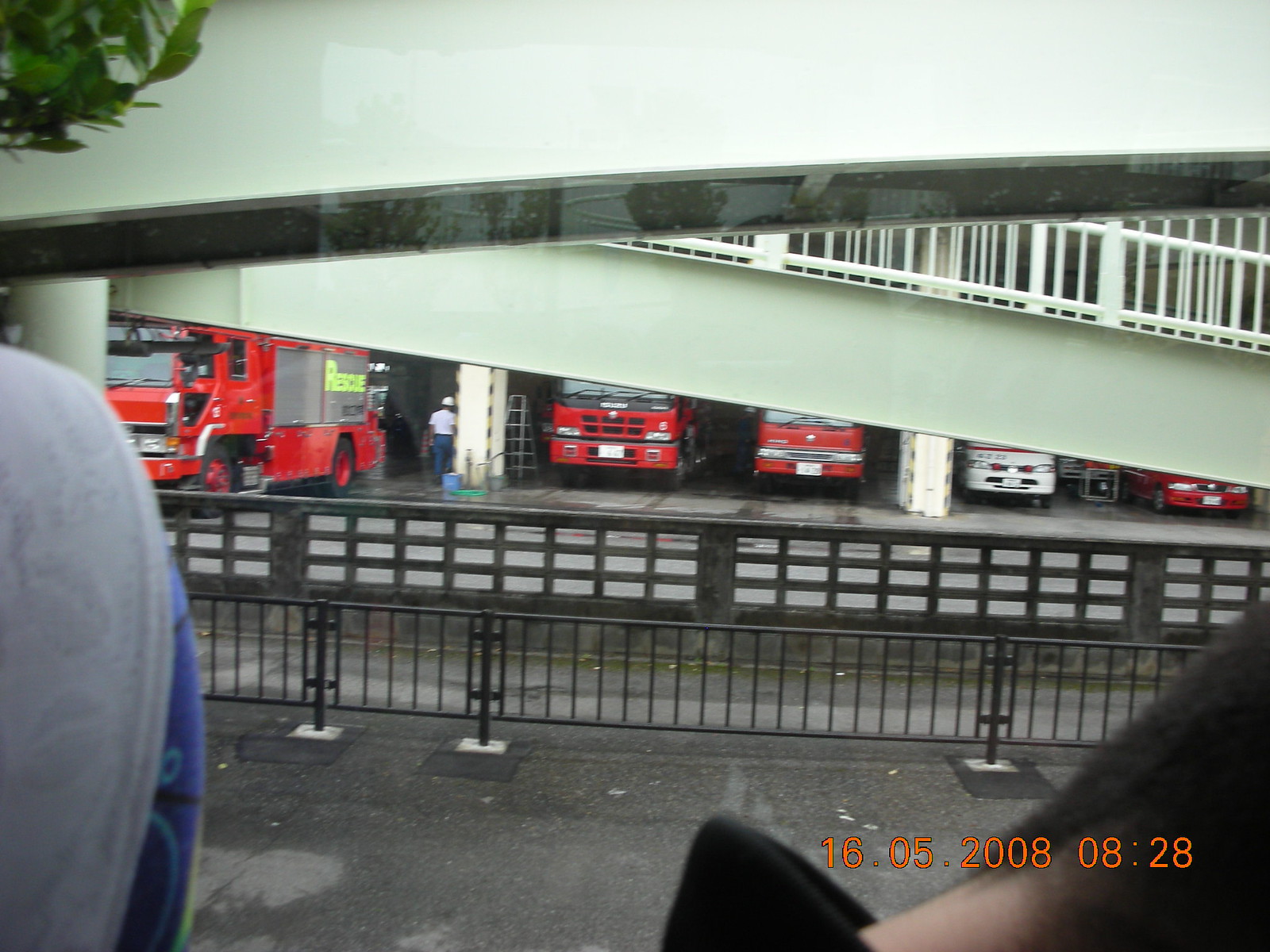In this detailed photograph taken on May 16th, 2008, at 8:28 in the morning, we see a fire station partially obscured by a lime-colored ramp and a concrete wall. The focal point is the array of fire trucks and service vehicles, some visible and some partially hidden within the bays of the station. On the left, a red fire truck is distinguishable beside a man dressed in blue denim jeans, a white t-shirt, and a hard hat. To his right are additional fire trucks, faintly visible behind a drive-up garage ramp. The image appears to be taken from a moving vehicle, likely a bus, as indicated by the blurred edges and the presence of a large reflective window. The scene is framed by low, dark fencing designed for crowd management, and in the bottom right-hand corner, a timestamp reads "1605 2008," marking the date and time of the photograph.